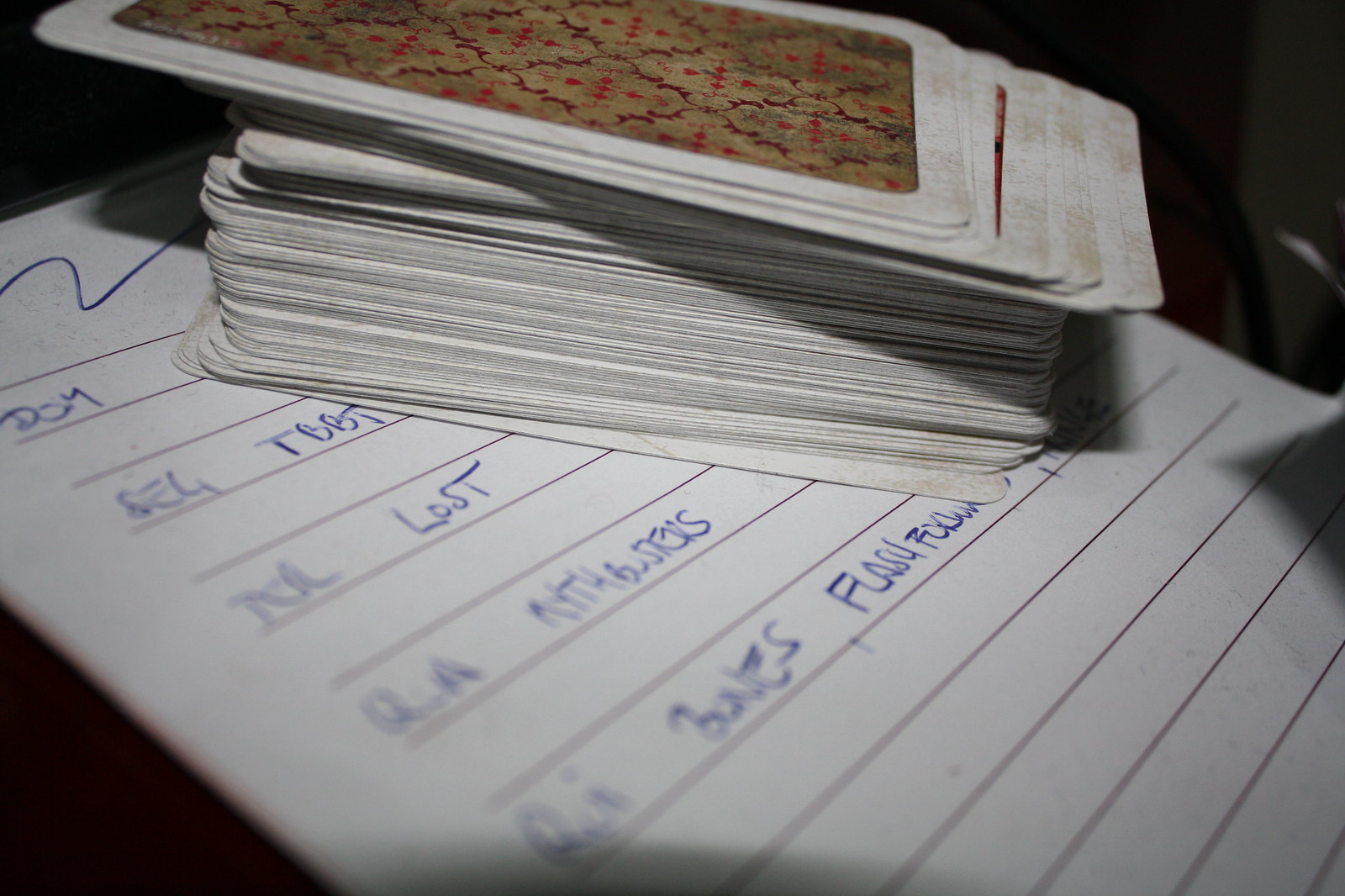A crisp white sheet of paper lies flat, its surface catching and reflecting the light in a way that highlights the horizontal lines printed across it. This lined paper resembles a typical notebook page. Written in blue ink on the paper is some text; however, it appears blurred, making the specific content indiscernible. Atop this sheet rests a deck of cards, meticulously stacked face down. The back of each card boasts an intricate, flowery design rendered in gold, red, and brown hues. The light source casts shadows on both the sheet of paper and the deck of cards, creating a subtle interplay of light and shadow across the scene.